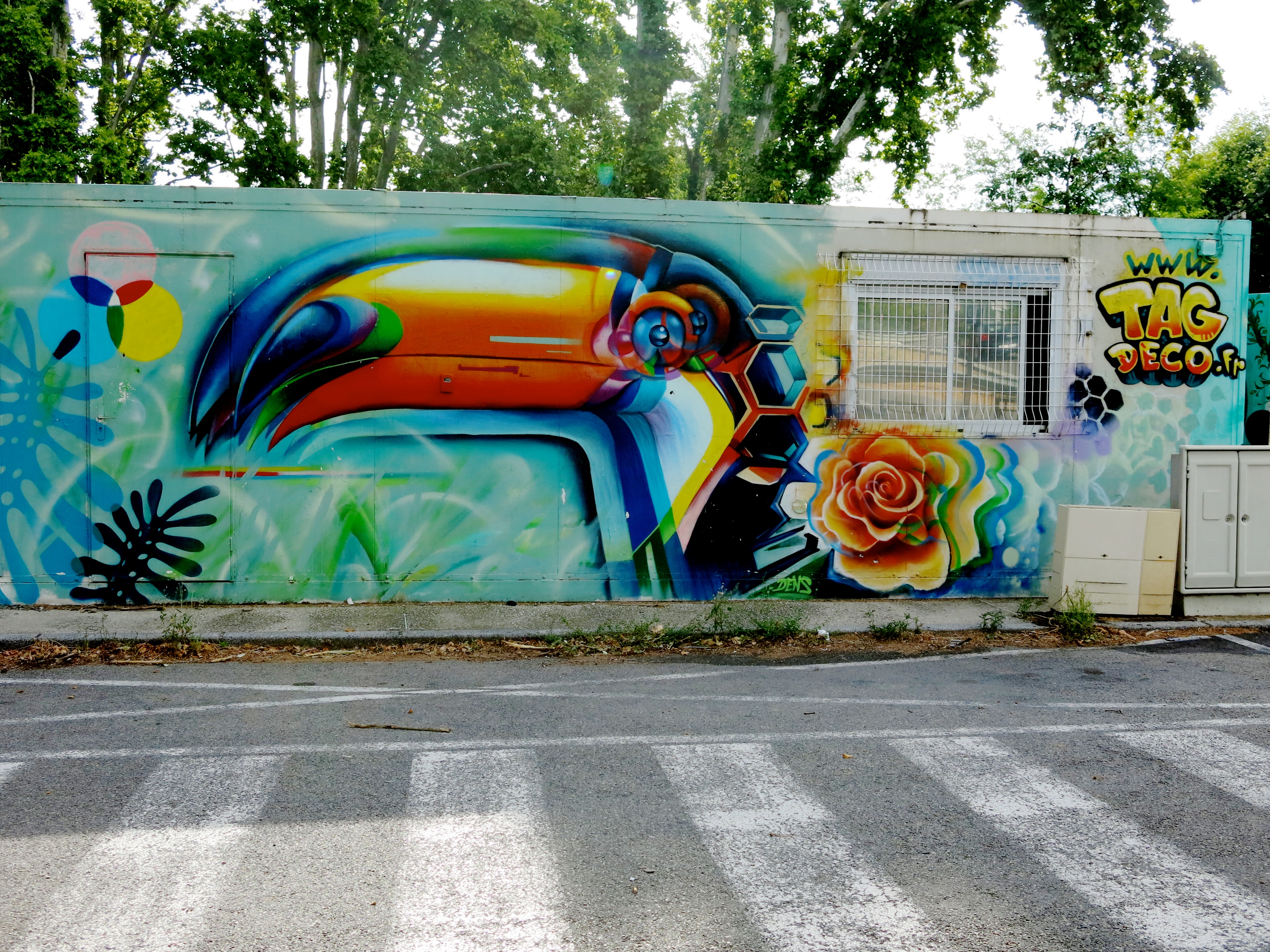The image depicts a large white mobile trailer centered on a cement slab with an asphalt parking lot in the foreground, marked by white painted stripes. The trailer is adorned with vibrant graffiti, featuring a toucan showcasing a striking palette of black, white, orange, green, and blue. The toucan, appearing to have two heads stacked vertically, looks toward the left side of the photograph. Surrounding the toucan's head are various leaves and ferns on the left, while an orange and yellow rose is painted to the right. Near the right side of the trailer, the graffiti includes the website "www.tagdeco.fr". Two storage cabinets sit in front of the trailer, and behind the scene, green trees stand against a pale sky. A window with netting is also visible on the trailer, adding to the eclectic details of the image.